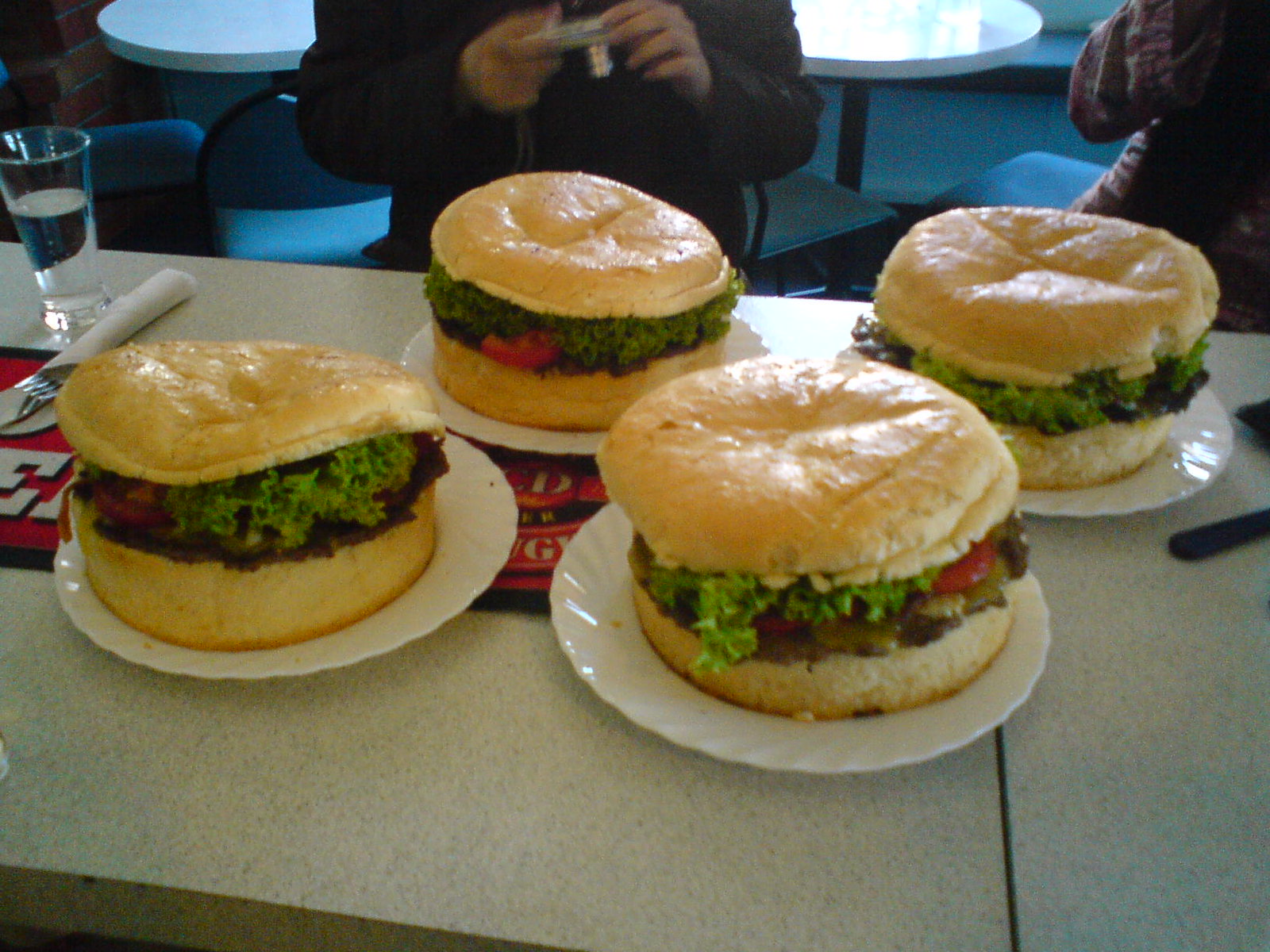The photograph captures a brightly lit restaurant setting, distinguished by shiny white Formica tabletops with chairs pulled up to them. Sunlight streams through a window, casting a bright glow on one of the tables. Centered on the table are four enormous hamburgers, each occupying an entire plate. These burgers feature thick bottom buns, thinner top buns, and are generously filled with lettuce, tomatoes, pickles, and a thin patty, with some of the toppings spilling out from the sides. A glass of water in a pilsner-style glass sits to the left of the frame, next to a neatly wrapped roll of silverware containing a knife and fork. Two people are partially visible in the background; one is wearing a black jacket and holding a camera, capturing the scene, while the other person, clothed in a jacket with loose sleeves, remains indistinguishable by gender. Their presence adds a candid, lived-in atmosphere to the diner environment.